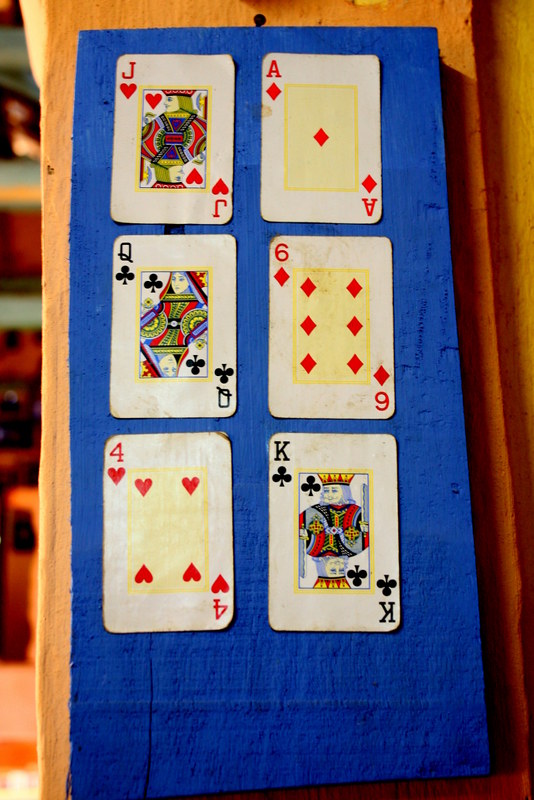In the image, a medium brown board serves as the backdrop, partially obscured by light blue and yellow shelving filled with various items, possibly toys. The focus is on a vibrant blue cloth draped over the brown board, displaying six playing cards arranged neatly in two columns and three rows. The cards include the Jack of Hearts, Ace of Diamonds, Queen of Clubs, Six of Diamonds, Four of Hearts, and King of Clubs. The setup casts soft shadows against the brown board. To the right, a yellow board is visible, adding contrast to the scene. The blue cloth has slight wrinkles, enhancing its rich, beautiful hue.